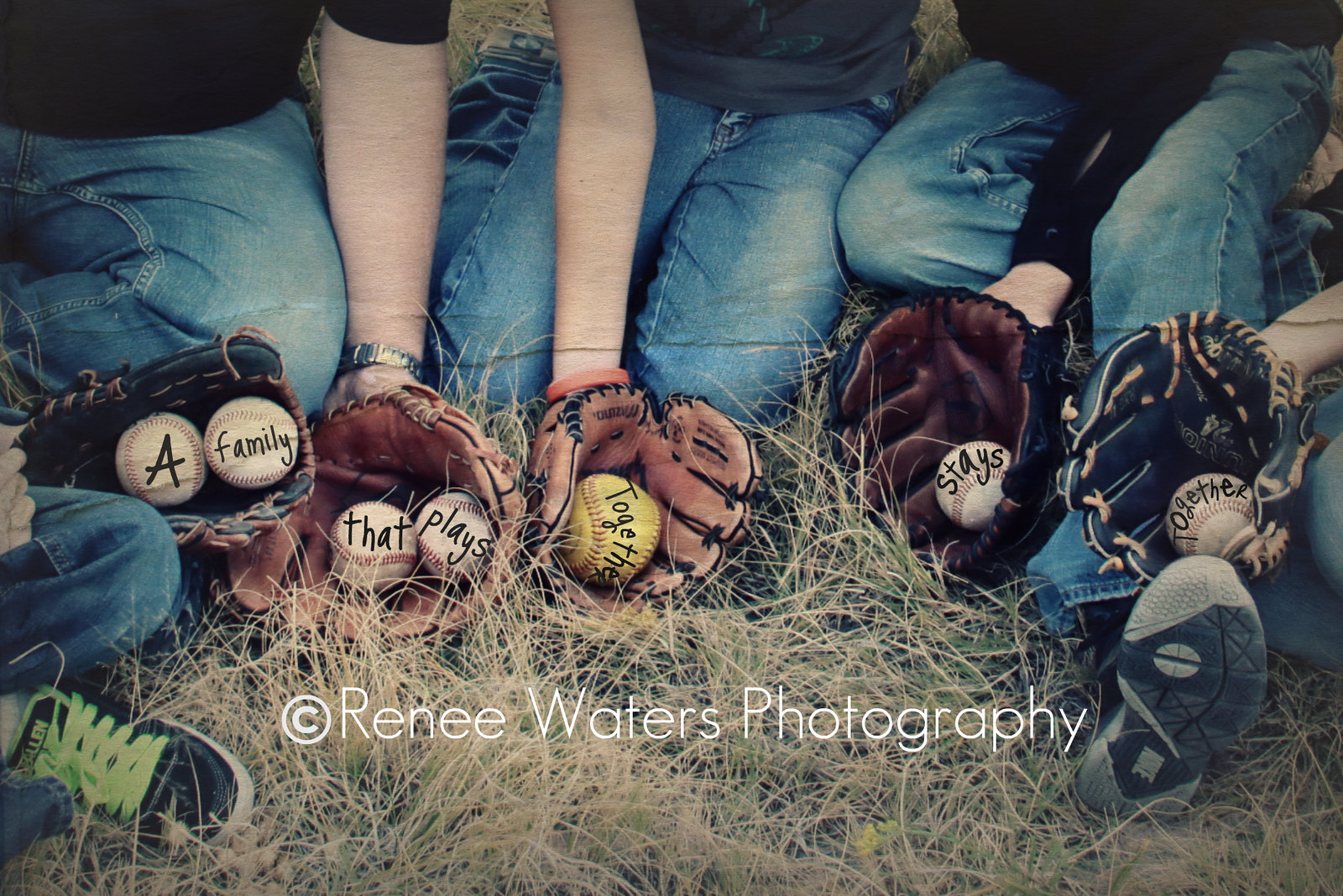The image is an advertisement for Rene Waters Photography, prominently featuring the copyright notice across the lower half in white text. It captures five people, presumably either children or family members, sitting on overgrown, slightly dead grass. Their identities are obscured as the photo only shows them from the waist down, revealing their blue jeans, dark tops, and a pair of fluorescent-laced trainers among regular shoes. Each individual wears a baseball mitt on their hand, each containing a baseball. From left to right, the baseballs spell out the phrase: "A family that plays together stays together," with one notably yellow baseball among predominantly white ones. The detailed arrangement and personal touches like a shiny wristwatch add to the intimate, homely quality of the photo.